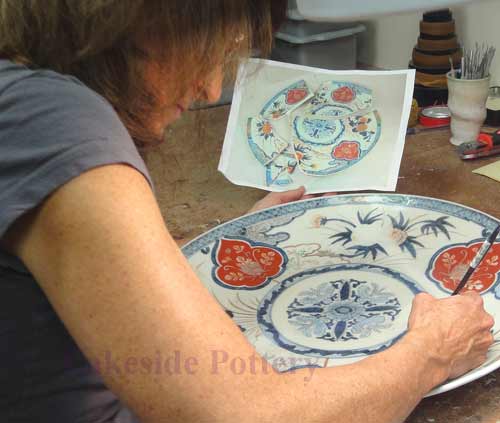In the image, a caucasian woman with brown hair, partially concealing her face, is captured while engaged in an artistic task. She is dressed in a gray T-shirt with partially obscured lettering on her arm that appears to read "Lakeside Pottery." She is working on a brown table and is holding up a white-framed picture. The picture features a patterned glass plate with a complex design. The plate displays a grey outer pattern, interspersed with white and blue outlines forming leaves. Within these outlines, red fills the inner spaces, accompanied by additional grey-patterned details. The central section of the plate exhibits a gradient pattern, transitioning from dark grey on the outermost ring to light white in the center, encircled by another greyish ring. Grey lines radiate towards the edge of the plate, transitioning into lighter grey with stem-like extensions emanating from the inner circle.